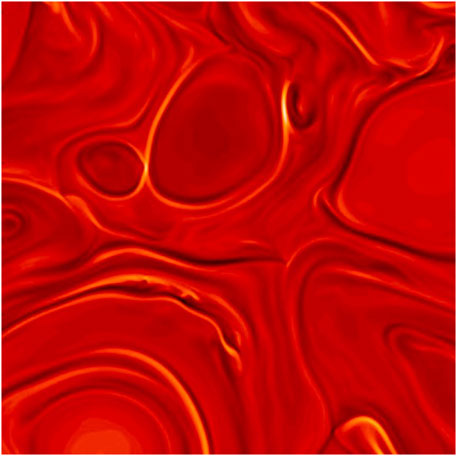This image presents a vivid, intricate piece of art that predominantly showcases red and orange hues, reminiscent of the colors of fire. The artwork appears to be computer-generated and contains various shapes and round figures, imbued with a consistent dark orange color. Some of these shapes are bordered by black and white hues. The overall composition is simple yet rich in texture, featuring circles of varying sizes and numerous intersecting lines, as if someone has drawn through the vibrant surface. Yellow rings and lines accentuate some of the red circles and indentations, adding depth and contrast. It evokes an impression of fluidity, as if capturing red liquid or paint in motion, displayed on a flat surface with intricate designs created by a brush. The striking use of bright red and detailed patterns gives the impression of a dynamic and textured creation, possibly a painting or a digitally rendered scene.